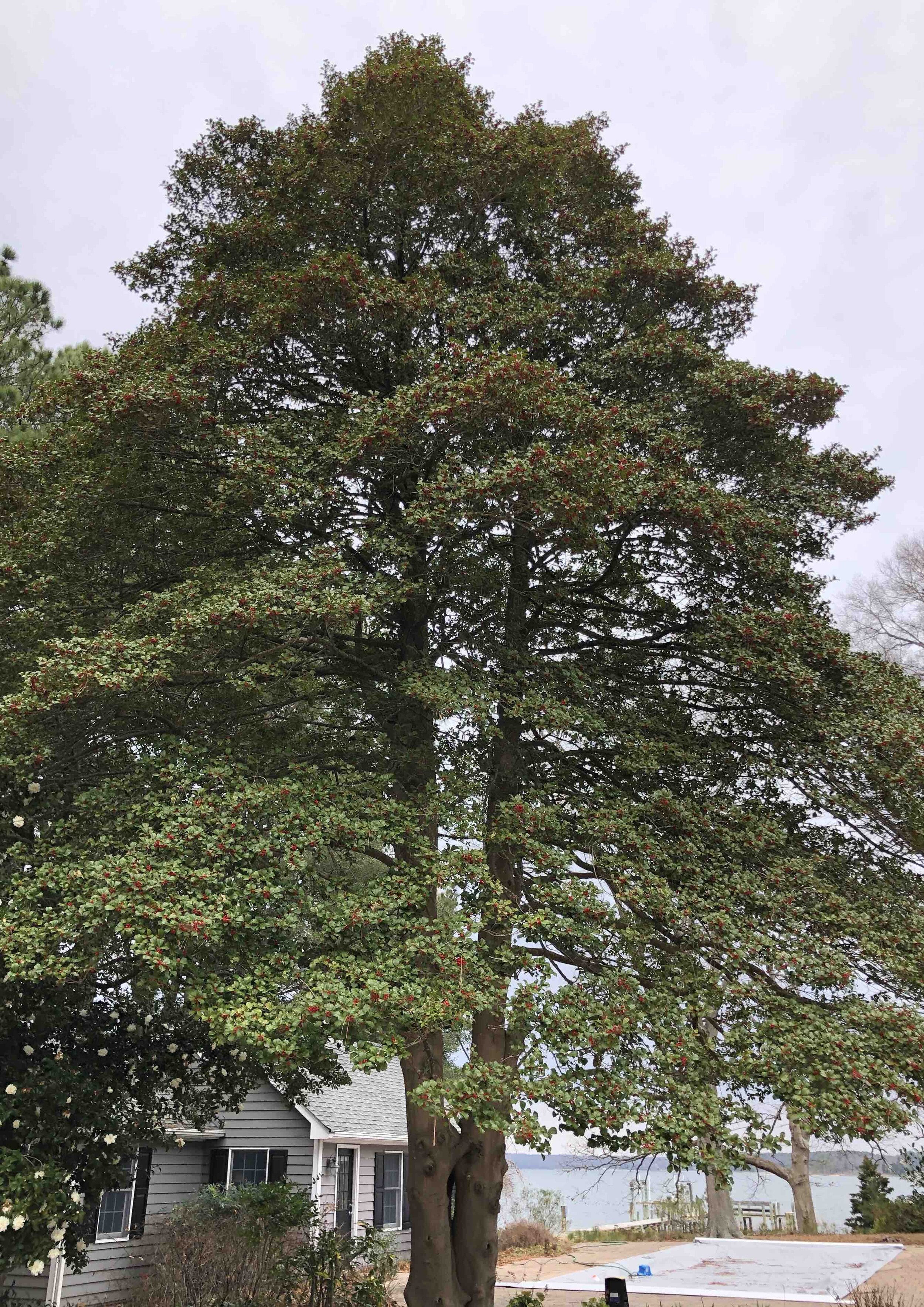This is a detailed photograph centered on a medium-sized tree with a unique shape, featuring a brown trunk that splits almost immediately into two thinner trunks. The foliage is dense with small, light green leaves that gradually darken toward the top, likely due to the varying sunlight. Interspersed among the leaves are numerous small red berries or flowers, adding vibrant color to the tree.

In the background, a single-story gray house with black-trimmed windows and a door is partially visible. In front of the house, there is a bush and another tree with white flowers. Further, to the right of the tree, a gravelly stone area with a tarp, possibly covering a pool, can be seen. Beyond the house and trees, there is a body of blue water, possibly a lake, with a bench nearby and mountains faintly outlined on the horizon under an overcast, gray sky, suggesting an impending storm.